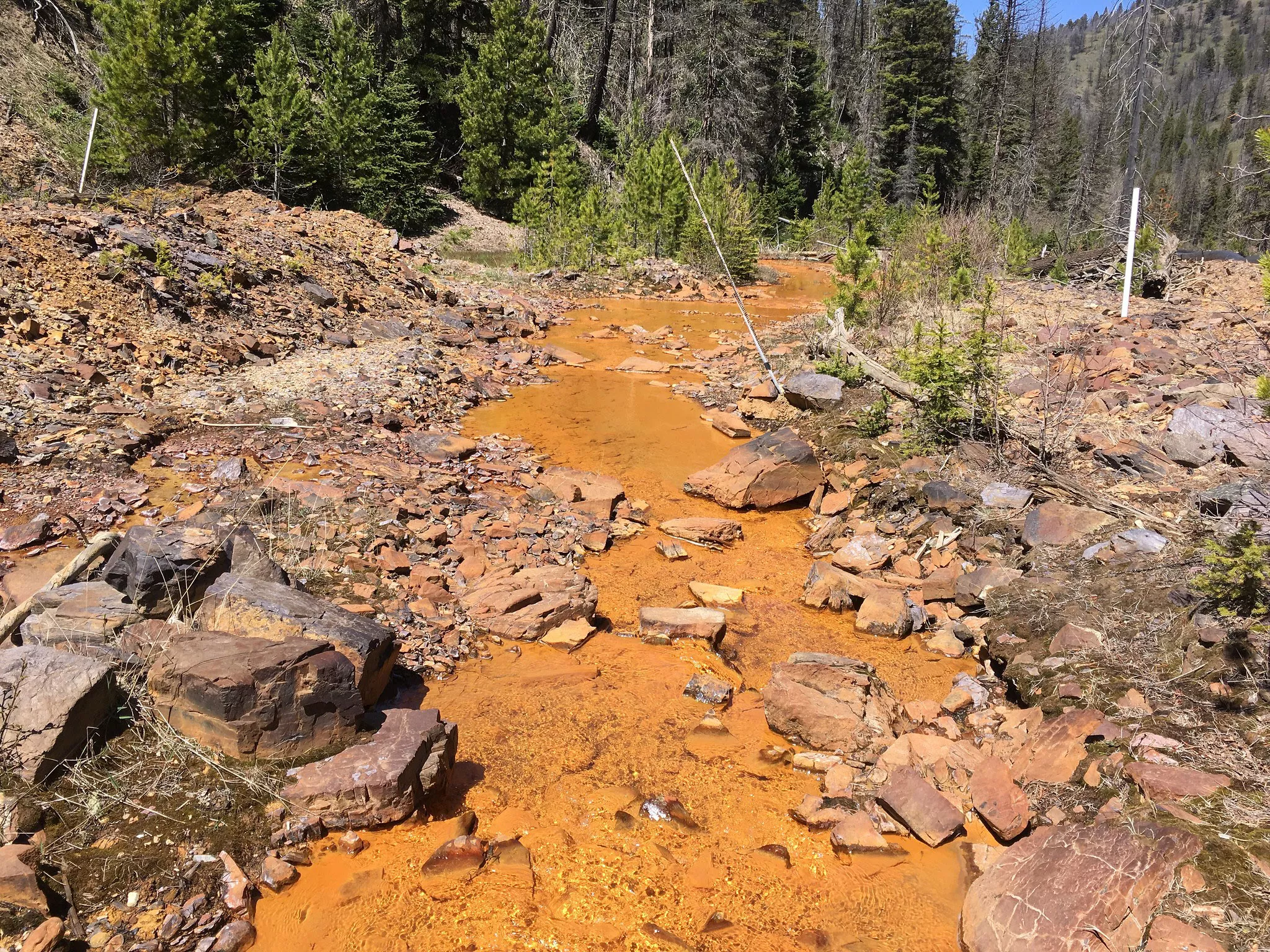A full-color photograph captures a serene yet troubled outdoor setting on a very sunny day. The scene appears to be from a western region, featuring a pine forest that is showing signs of distress, with many pine trees standing bare. Dominating the foreground is a dried-up riverbed, its course marked by flat, shale-like rocks. These rocks are contrasted by the golden-brown hue of the riverbed itself, suggesting the recent presence of water. Winding through the lower part of the image is a narrow stream with distinctive orange-colored dirt, making sharp turns as it meanders towards the center. The stream is flanked by numerous rocks in varying shades of rust, gray, and brown, cluttering its banks. As one's gaze moves towards the background, the scene transitions to patches of greenery, with clusters of healthier trees on the left and more distressed pines stretching off into the horizon.